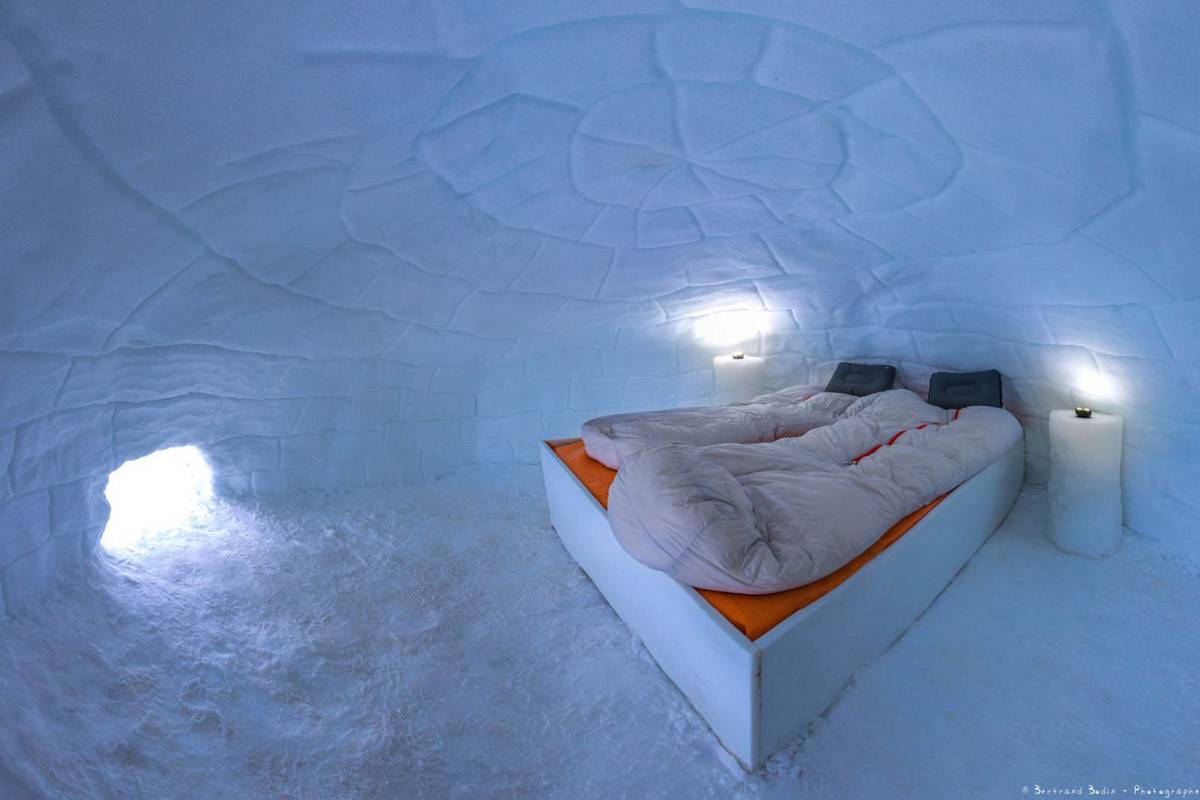The photograph showcases the interior of an igloo, meticulously constructed from blocks of snow with a snow floor. The spacious, snowy igloo has a small entrance hole at the bottom right, through which sunlight pours in. Central to the scene is a white platform bed with an orange mattress, accompanied by two tan sleeping bags, each equipped with a colorful zipper. Two gray pillows rest against the headboard. Flanking the bed on either side are white, oval-shaped bedside tables that resemble the shape of tree stumps, each bearing a small light on top, casting a subtle glow that highlights the textured ice construction. The caption at the bottom right corner reads "Bertrand Bowden Photographer."